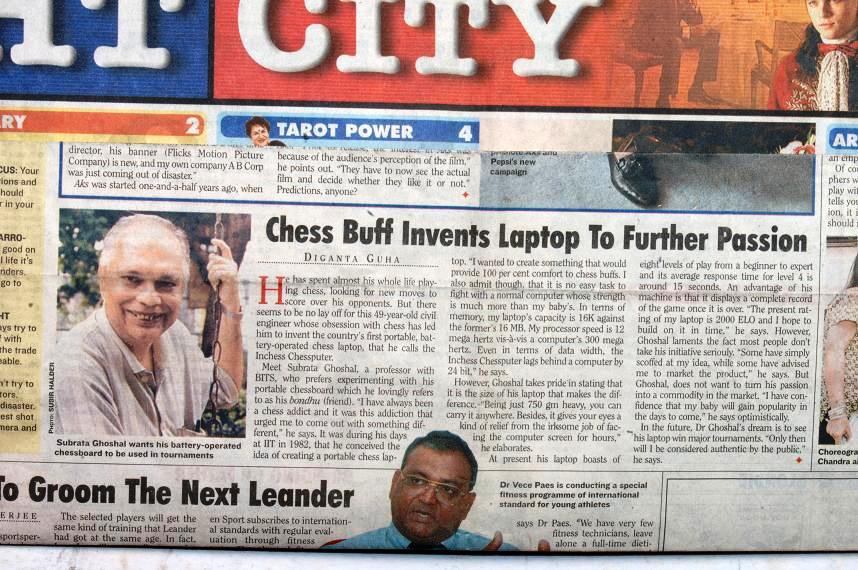In this newspaper clipping, the front page prominently features an article titled "Chess Buff Invents Laptop to Further Passion," authored by Diganta Guha. Central to the page is a photograph of an elderly man, likely in his late 60s, smiling as he sits on a swing set. He is dressed in a white-collared shirt adorned with stripes and has thinning white hair. The caption beneath his image identifies him as Subrata Goshal (spelled S-U-B-R-A-T-A G-H-O-S-H-A-L) and notes that he wants his battery-operated chessboard to be used in tournaments. Above this main article, there's mention of "Tarot Power" on page number four. The page is also accented with a blue rectangle to the top right and an orange one to the top left, partially displaying the words "city" and "T" respectively. Below the main article, another photograph depicts a man with a mix of black and white hair, wearing glasses. He appears to be South Asian and is associated with the title "Groom the Next Leander."